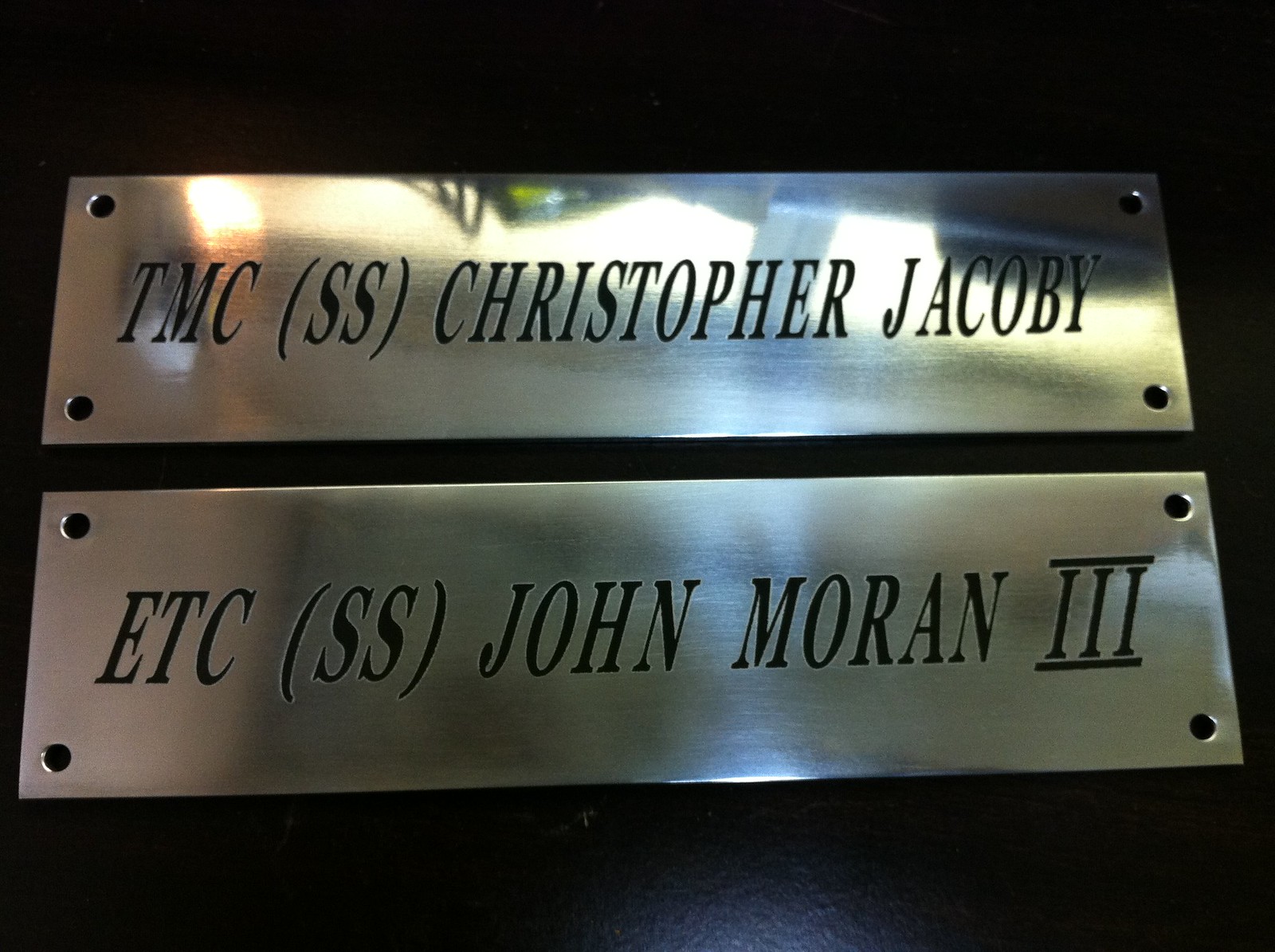The image showcases two rectangular metallic nameplates, each featuring four indentations at the corners for mounting, likely with screws. Both nameplates are aligned side by side on a dark, possibly black, table. The first nameplate, adorned with a gold-like or silver finish, reads "TMS (SS) Christopher Jacobi" in black engraving. The second, identical in shape and color, reads "ETC (SS) John Moran III." The metallic surfaces reflect ambient details of the room, emphasizing their lustrous appearance. Overall, the intricate design and the reflection on the nameplates hint at a polished, formal setting, possibly for a door or a commemorative plaque.